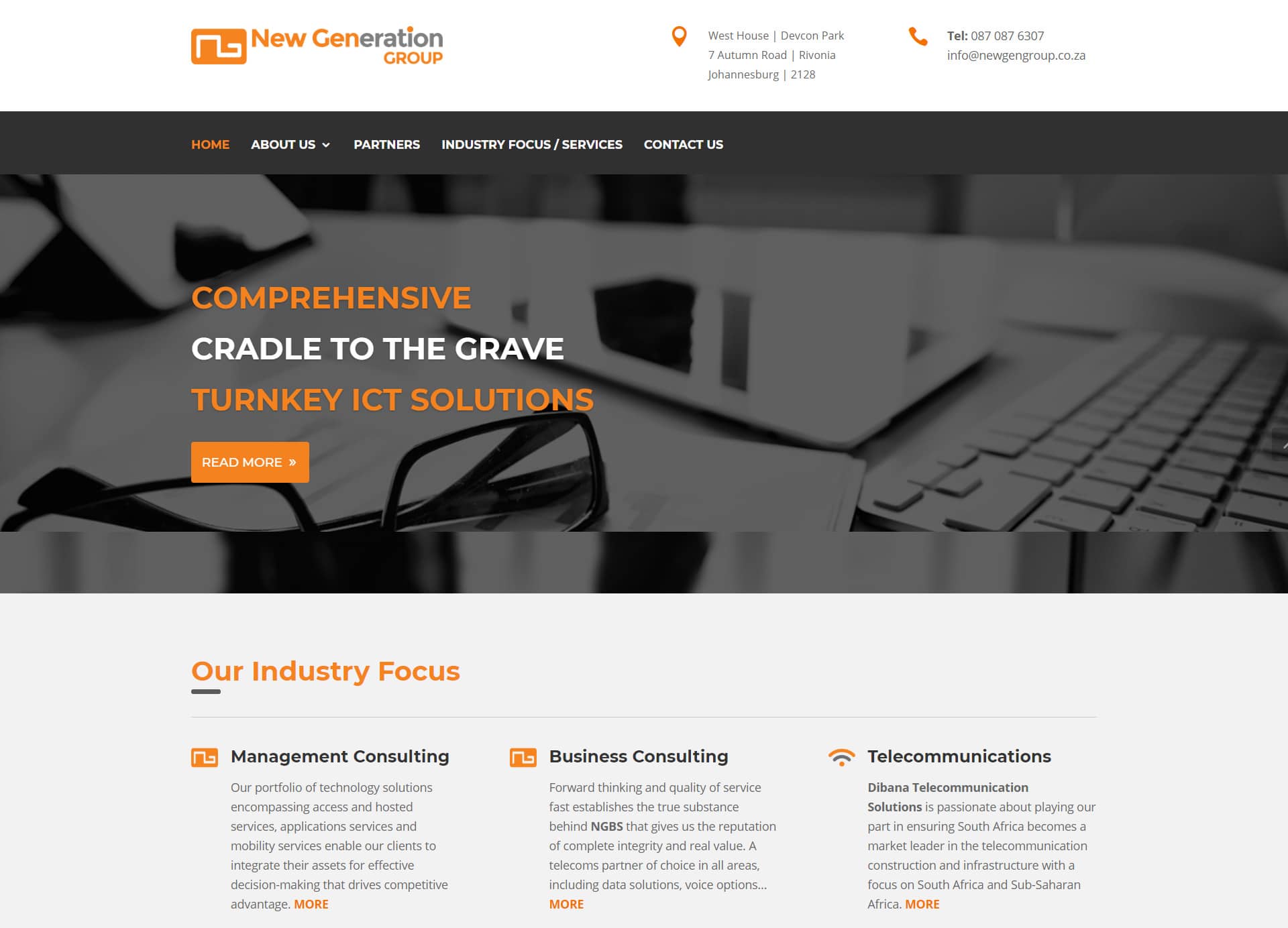**Detailed Image Caption:**

In the top left corner of the image, the text "New Generation Group" is prominently displayed, featuring white letters against an orange background, with the word "Group" highlighted in purple. Moving to the right, the image includes both the address and contact information of the organization.

The primary focus of the image is a central design characterized by a mix of gray and black colors. Dominating this section, the phrase "Comprehensive, cradle to the grave, turnkey ICT solutions" is arranged strategically. "Comprehensive" is highlighted in orange, the words "cradle to the grave" appear in white, and "turnkey ICT solutions" reverts back to orange. Below this text, a "Read more" prompt is evident, with the text in white against an orange background.

The overall color scheme employs a light gray dominance, interspersed with different colors for emphasis. A noteworthy design element in the center includes an image resembling a pair of glasses to the left and a light gray keyboard on the right. Some sections of black are integrated on the left side of this central design, complementing the predominant gray.

Towards the bottom, the background lightens considerably, and the text "Our Industry Focus" is written in orange. Below this header, three distinct sections are clearly labeled: "Management Counseling" on the left, "Business Consulting" in the middle, and "Telecommunications" on the right. Each section is accompanied by an icon on its left side and a paragraph of gray text below it. Each paragraph concludes with the word "More" highlighted in orange.